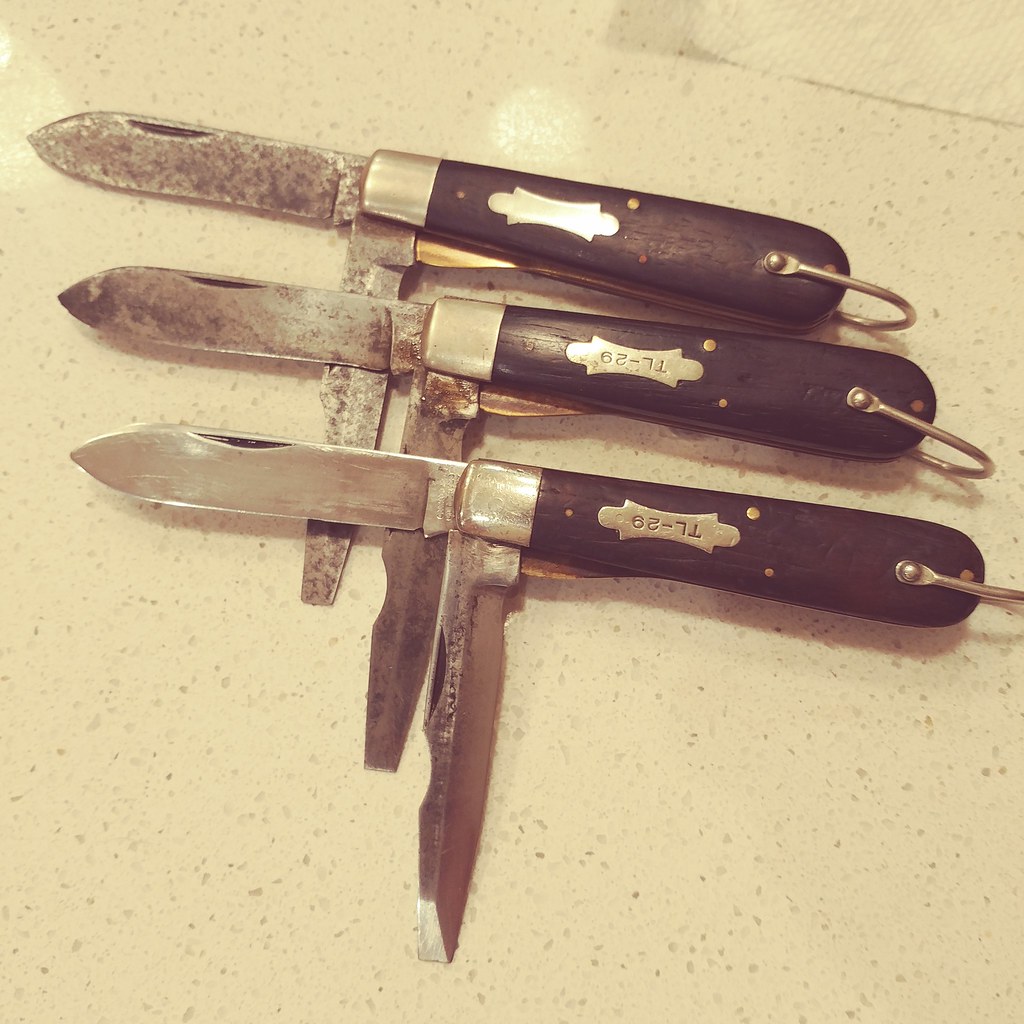A detailed photograph showcases three vintage pocket knives meticulously arranged in a row on a white granite-like countertop, speckled with gray and black dots. Each knife is positioned with its main blade extending straight out to the right, while an additional blade points downward, forming a distinctive T shape. The two knives at the back display considerable rust on both blades, while the foremost knife has a clean main blade but a slightly rusty smaller blade. All three knives feature black, tapered wooden handles adorned with a few shiny silver rivets and a silver metal guard where the blades fold. Each handle also includes a metal loop at the end, suitable for attaching to a key ring. Notably, the handles of two of the knives bear the inscription "TL-29" in a silver emblem, adding a unique historical detail to their appearance. In the top right corner of the image, a piece of white napkin paper is partially visible, adding a touch of context to the setting.